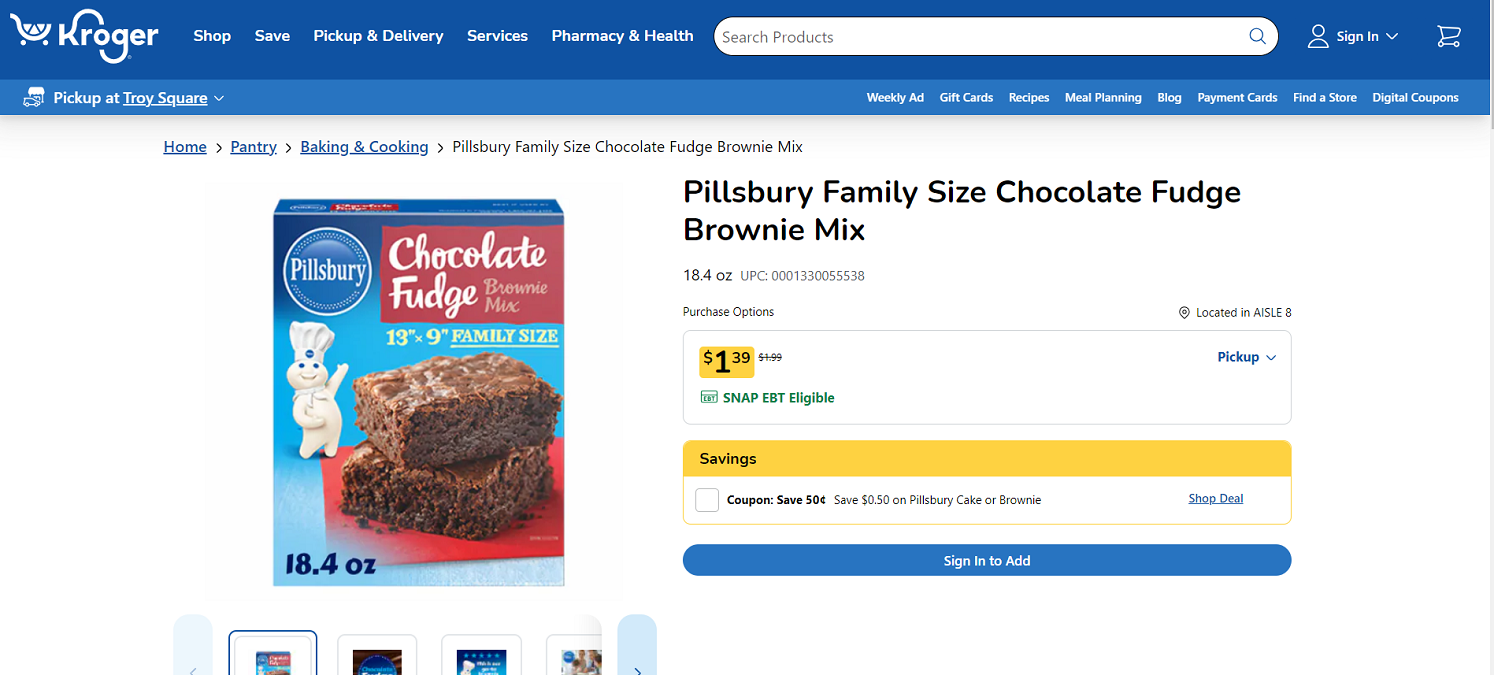The image depicts a capture of the Kroger supermarket website. In the upper left corner, the Kroger logo is prominently displayed beside a shopping basket icon. A blue navigation bar extends across the top of the page, featuring options such as "Shop," "Save," "Pickup & Delivery," "Pharmacy," and "Health."

Below this navigation bar, there is a search bar for finding products. On the right side, you can sign in to your account or add items to your cart. There's also a specific pickup location indicated as "Choice Square."

Underneath, several shopping categories are listed, including "Home," "Pantry," "Baking," and "Cooking," all highlighted in blue. A detailed product feature occupies a significant portion of the page, showcasing Pillsbury Family Size Chocolate Fudge Brownie Mix. The product name is displayed in light black print, accompanied by an image of the brownie mix box. The box features the Pillsbury Doughboy and an image of two rich, chocolate brownies stacked on top of each other. This family-sized box, weighing 18.4 ounces, is designed for a 13x9-inch pan.

To the right of the product image, there is a detailed description including the price of $1.39, a note that it is SNAP EBT eligible (marked in green), and the Universal Product Code (UPC) symbol. There is an option to pick up the item, indicated by a drop pin icon. Additionally, a savings banner runs across, highlighted in gold, mentioning a 50-cent coupon which requires signing in to apply.